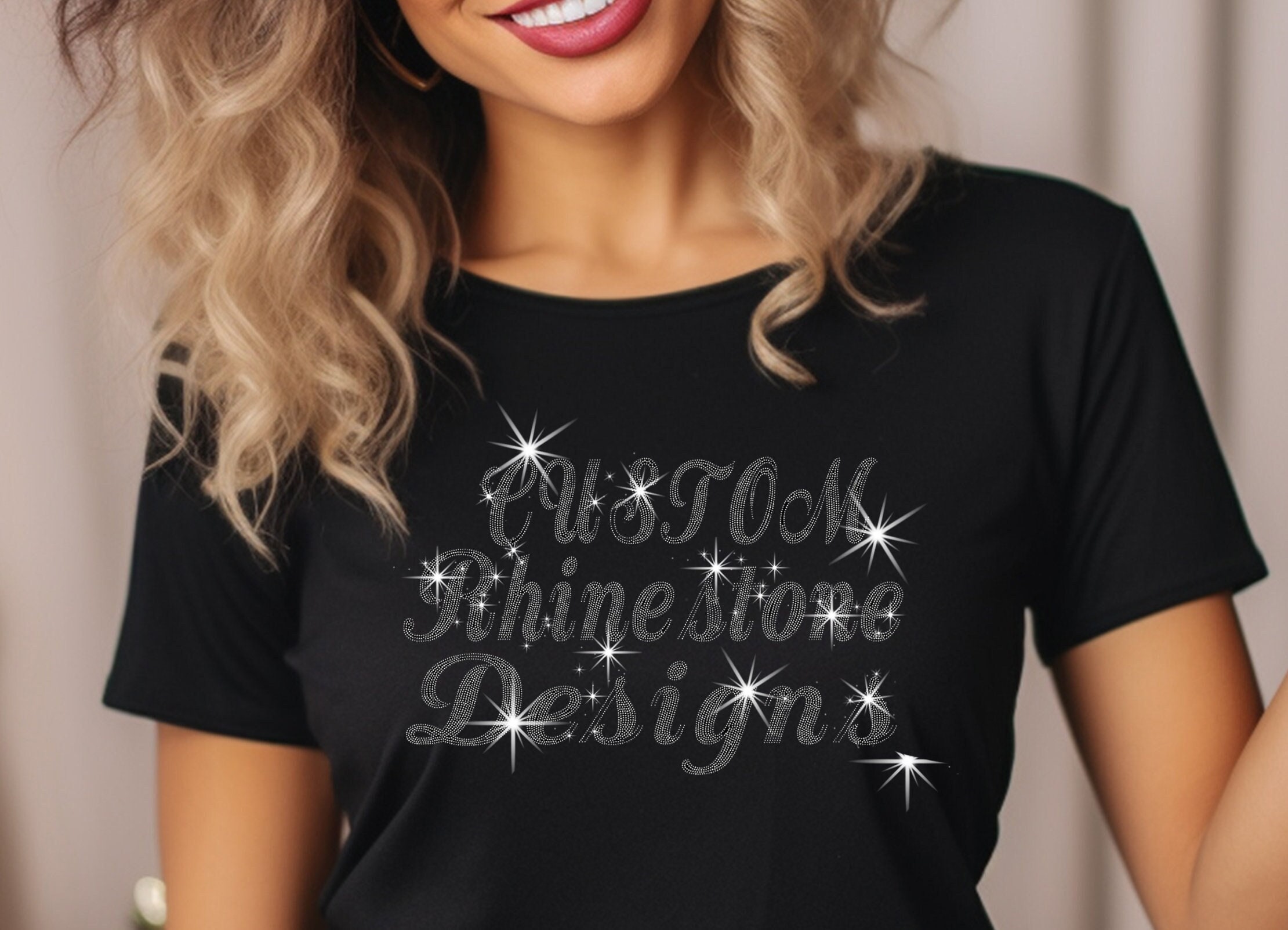This photograph features a young woman with curly, blonde hair tinged with brown that cascades just past her shoulders. Her light-colored skin radiates against a plain white background, which accentuates her vibrant red lips and beaming white teeth, visible halfway as her head is tilted slightly to the left. The image is cropped from the middle of her mouth downward to just above her waist, revealing her black short-sleeved t-shirt. The shirt is adorned with a fancy calligraphic design that reads "custom" with "rhinestone designs" beneath it, both phrases punctuated by sparkling rhinestones that mimic bright white stars. Her right arm hangs naturally by her side while her left arm bends up slightly and extends out of the frame.